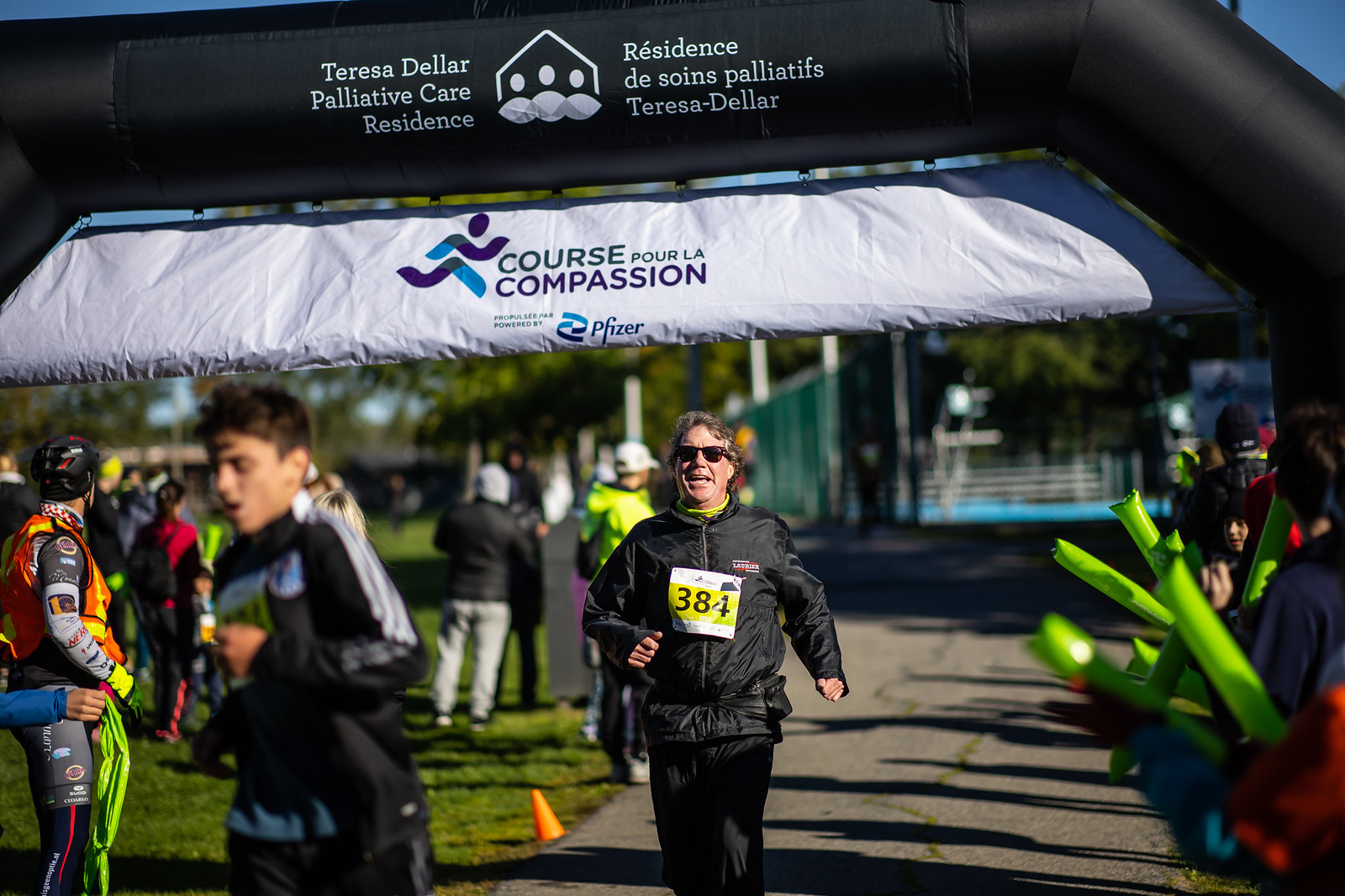The photograph captures a charity race event held under a large black blow-up archway that reads "Teresa Deller Palliative Care Residence." Below the archway, a white banner displays "Course Compassion" with a runner logo and an advertisement for Pfizer. In the foreground, a younger boy is partially out of focus, dressed in a black windbreaker with white stripes, jogging on a cement road. Prominently in focus is an older gentleman wearing sunglasses, also in a black jogging suit, running with a yellow tag featuring the number 384 pinned to his jacket. Surrounding the race pathway, several people cheer on the participants, many holding green inflatable noisemakers. The background showcases a grassy area with trees and possibly a swimming pool or tennis courts, adding context to the lively atmosphere of the event.